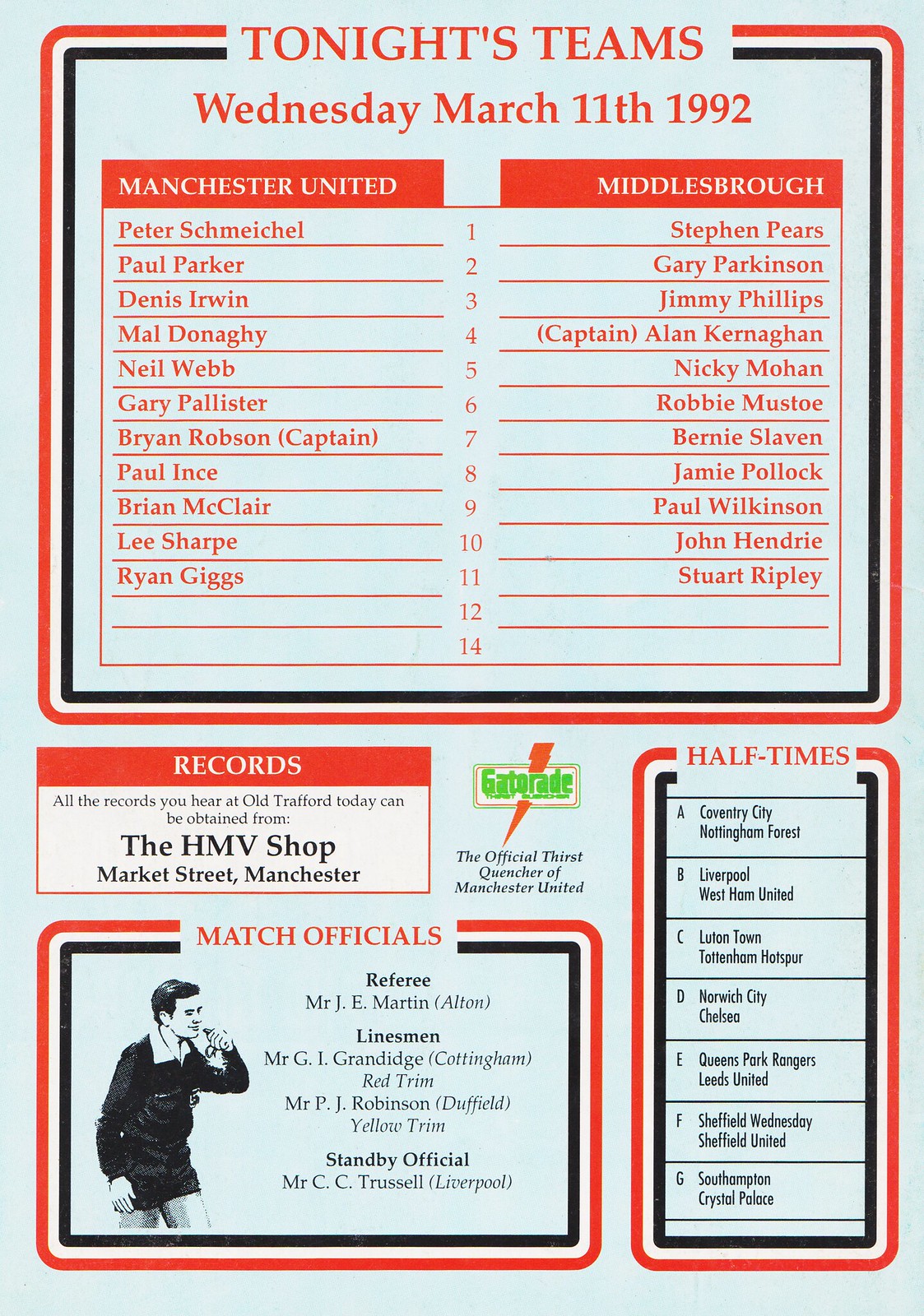The image is of a detailed football match information sheet with a light blue background, bordered in red, white, and black. At the top, bold red text reads "Tonight's Teams" followed by "Wednesday, March 11, 1992." The sheet features two columns listing the teams: Manchester United in white letters over red and Middlesbrough in white letters over a red bar. Each team's roster includes the players' names and numbers, such as Peter Schmeichel (1), Paul Parker (2), and Bryan Robson (7) for Manchester United, while Middlesbrough's list starts with Stephen Pears (1). A red bar at the bottom of the columns reads "Records" with a note about obtaining records from "The HMV Shop, Market Street, Manchester." Below this is an ad for Gatorade in green and orange, proclaiming it as the official thirst quencher of Manchester United. On the right, a skinny rectangle details "Halftimes" and "Match Officials," including referee Mr. J. Martin from Alton and linesmen Mr. G.I. Grandridge from Cunningham and Mr. P.J. Robinson from Duffield. At the sheet's bottom are small text areas providing additional details about match officials, illustrated with a drawing of a man in black with a whistle.